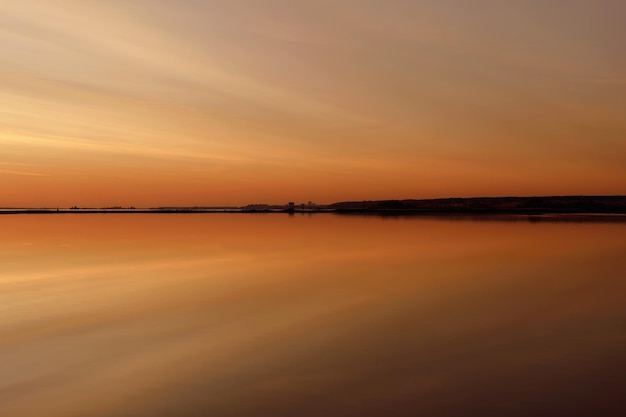The image features a serene waterscape at either sunset or dusk, with the viewer positioned in the middle of a perfectly still body of water, looking towards a distant, dark shoreline. The composition is strikingly symmetrical, as the sky is impeccably mirrored on the water's surface, creating an almost surreal, reflective effect. The sky is a complex tapestry of cloud streaks, primarily in shades of rich orange, yellow, gold, peach, and violet, making it devoid of the typical blue hues. These streaks stretch diagonally from the top left to the bottom right, intensifying the dusk-like atmosphere. The horizon line is marked by a flat, black landmass that divides the image into two equal halves, enhancing the mirror image effect. The scene is devoid of any wildlife, emphasizing the tranquil and peaceful quality of the moment captured.